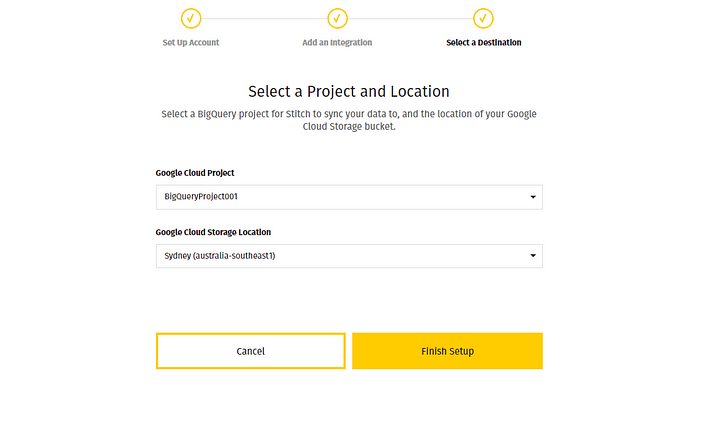The screen print depicts the setup progress bar at the top, featuring three yellow check marks situated at the beginning, middle, and end, each circled for emphasis. Below the first check mark, the text reads "Setup Account" in gray. The middle check mark is accompanied by the text "Add an Integration," also in gray. The final check mark aligns with the bold black text "Select a Destination." 

Directly beneath the progress bar, in larger font, is the instruction "Select a Project and Location." Following that, in smaller font, the text states, "Select a BigQuery Project for Stitch to sync your data to, and the location of your Google Cloud Storage bucket."

The section for selecting a project is highlighted with the bold label "Google Cloud Project." This is accompanied by a rectangular dropdown window displaying the selection "BigQuery Project 001." 

Next, under the bold label "Google Cloud Storage Location," there is another rectangular box showing the selected location, "Sydney," followed by "(Australia-Southeast1)" in lowercase.

At the bottom, there is a white rectangular button outlined in yellow, featuring black text that reads "Cancel." Directly next to it is a yellow rectangular button with black text that states "Finish Setup."

The layout is meticulously organized to guide users through setting up their project and location in Google Cloud, ensuring clarity and ease of use.